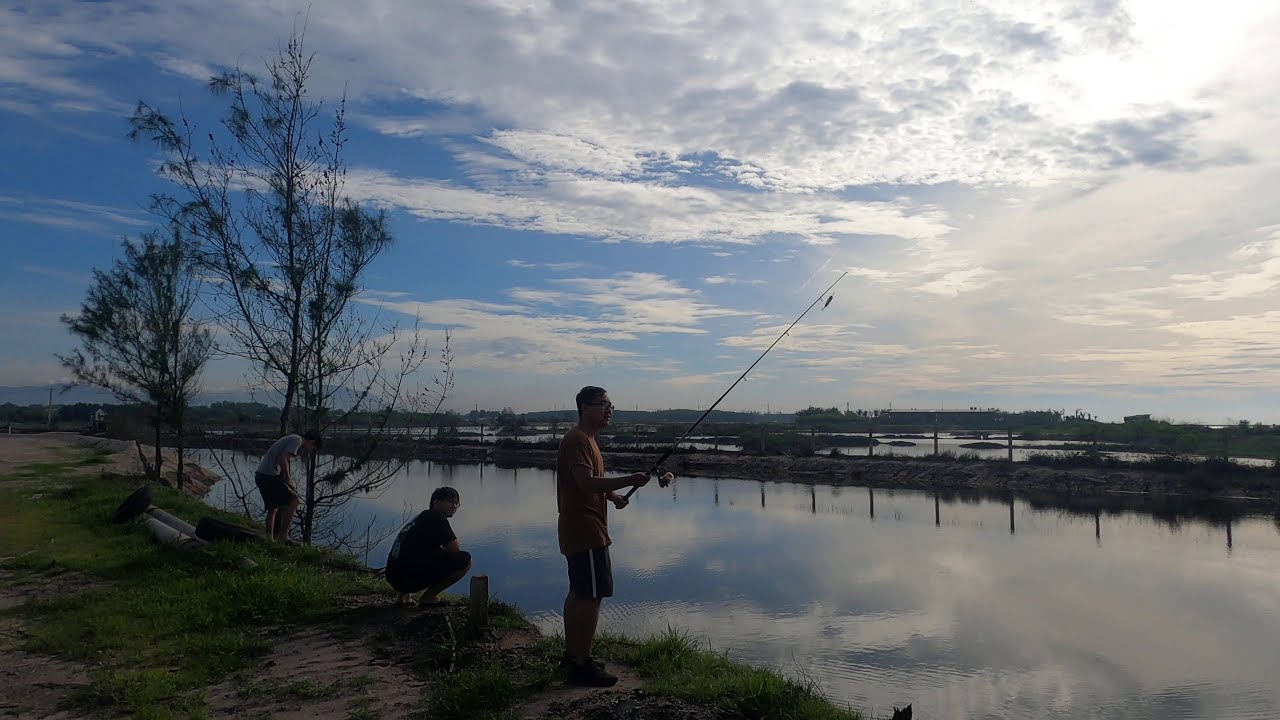This horizontally aligned rectangular picture captures a tranquil outdoor scene dominated by a vibrant sky that occupies the upper half. The sky is a picturesque blend of blue with gray puffy clouds and delicate white feathery clouds, with sunlight streaming in from the upper right-hand corner, lending a radiant glow to the image. 

In the foreground, a man stands in a grassy dirt area, facing towards the right. He is holding a fishing pole and is dressed in a short-sleeve brown or orange shirt paired with athletic shorts. To his side, another man wearing a black short-sleeve shirt and shorts kneels on the ground, looking up at him. On the left side, a third man in a white short-sleeve shirt and black shorts is peering down over the bank into the water. 

The water below is notably calm, with gentle ripples softly distorting the grayish-blue surface that captures reflections of the cloudy sky above. In the distance, a dock or man-made strip of land divides the water into sections, marked by a post-like fence. The setting exudes a serene, midday atmosphere perfect for fishing by a tranquil lake, framed by the gentle hues of green, brown, yellow, blue, gray, white, and black.